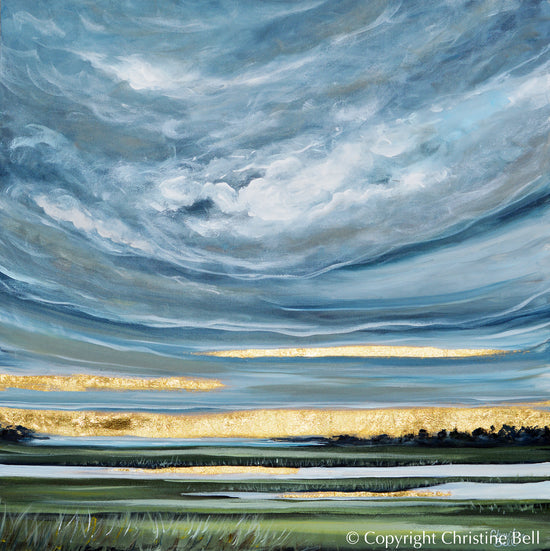This image is a computer-generated artwork or potentially a real painting or photograph by Christine Bell, as indicated by the copyright symbol in the bottom right corner. The scene depicts a dramatic outdoor landscape with an expansive sky taking up the majority of the frame, characterized by swirling clouds in shades of blue, gray, charcoal, gold, and yellow. The foreground features a patch of grass on the bottom left, while the background reveals a subtle hint of a forest. There may also be elements that suggest a stream, snow, or sand, adding to the diverse textures and colors seen in the image. The overall composition emphasizes the vastness of the sky and its dynamic cloud formations, creating a sense of an impending or recently passed storm.